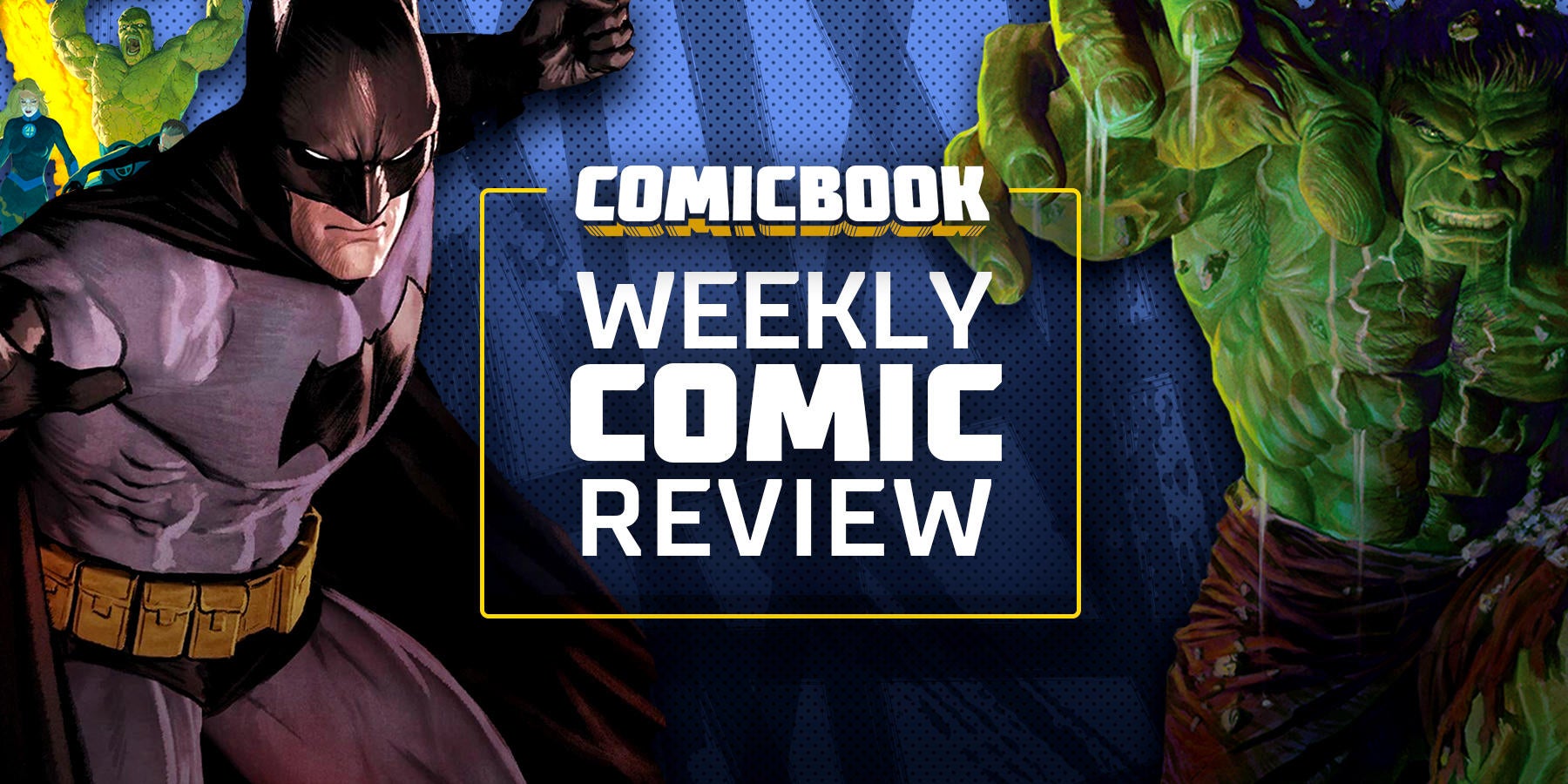This advertisement is a vibrant, colored graphic drawing formatted as a long rectangle. At the center, white letters outlined by a yellow box prominently display "comic book" at the top and "weekly comic review" beneath it. On the left side of the image is a fierce and aggressive Batman, adorned in his signature black cowl, black gloves, and a gray skintight suit with a black bat emblem on his chest. He also sports a gold utility belt and a black cape. Batman's left hand is clenched into a fist, while his right arm is extended as if he is mid-action in a fight. Behind him, partially obscured, are two characters: a green monster reminiscent of a less impressive Hulk and a woman whose details are less defined.

On the right side, the Hulk dominates, his green muscular form clad in brown pants. He leans forward menacingly, with one arm reaching towards the text, looking as if he's about to engage in combat. The background features a blue color scheme with darker blue stripes that add to the overall comic book aesthetic.